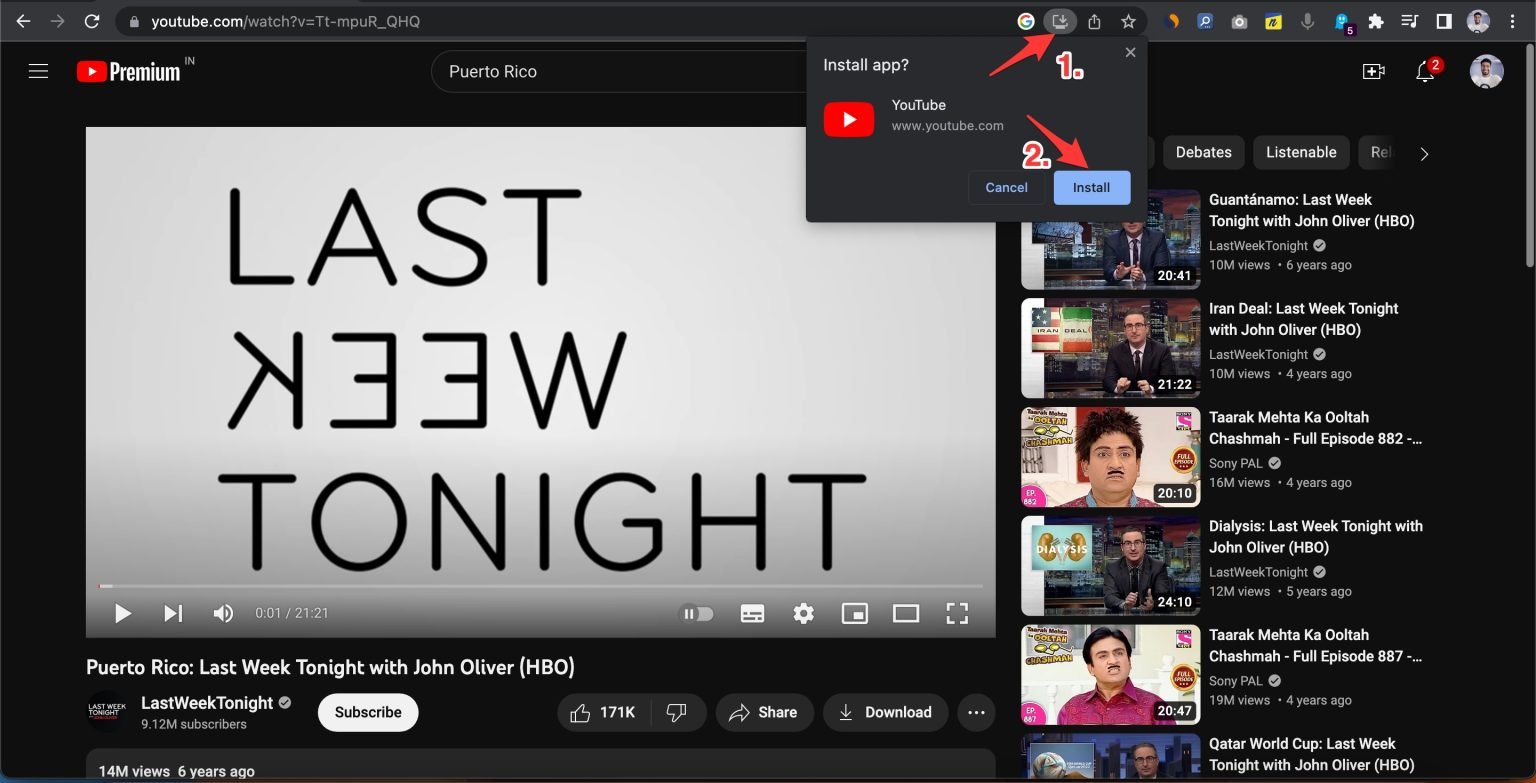The image features a section of a web browser displaying YouTube. In the top-right corner, there is a small box containing several icons, as well as a URL bar with a YouTube address. A pop-up window is visible, prompting the user to "Install app: youtube.com," accompanied by a blue "Install" button and a "Cancel" button beside it.

The main content of the screen shows a YouTube video titled "Last Week Tonight," with the subtitle "Puerto Rico: Last Week Tonight with John Oliver on HBO." Below the video, there is a prominent white "Subscribe" button. To the right of the main video, there is a list of recommended videos, including titles such as "Guantanamo: Last Week Tonight with John Oliver," "Iran Deal: Last Week Tonight with John Oliver," "Dialysis," and "Qatar World Cup."

In the upper-right corner, the notification bell icon indicates there are three notifications, and a profile picture is visible to its right.